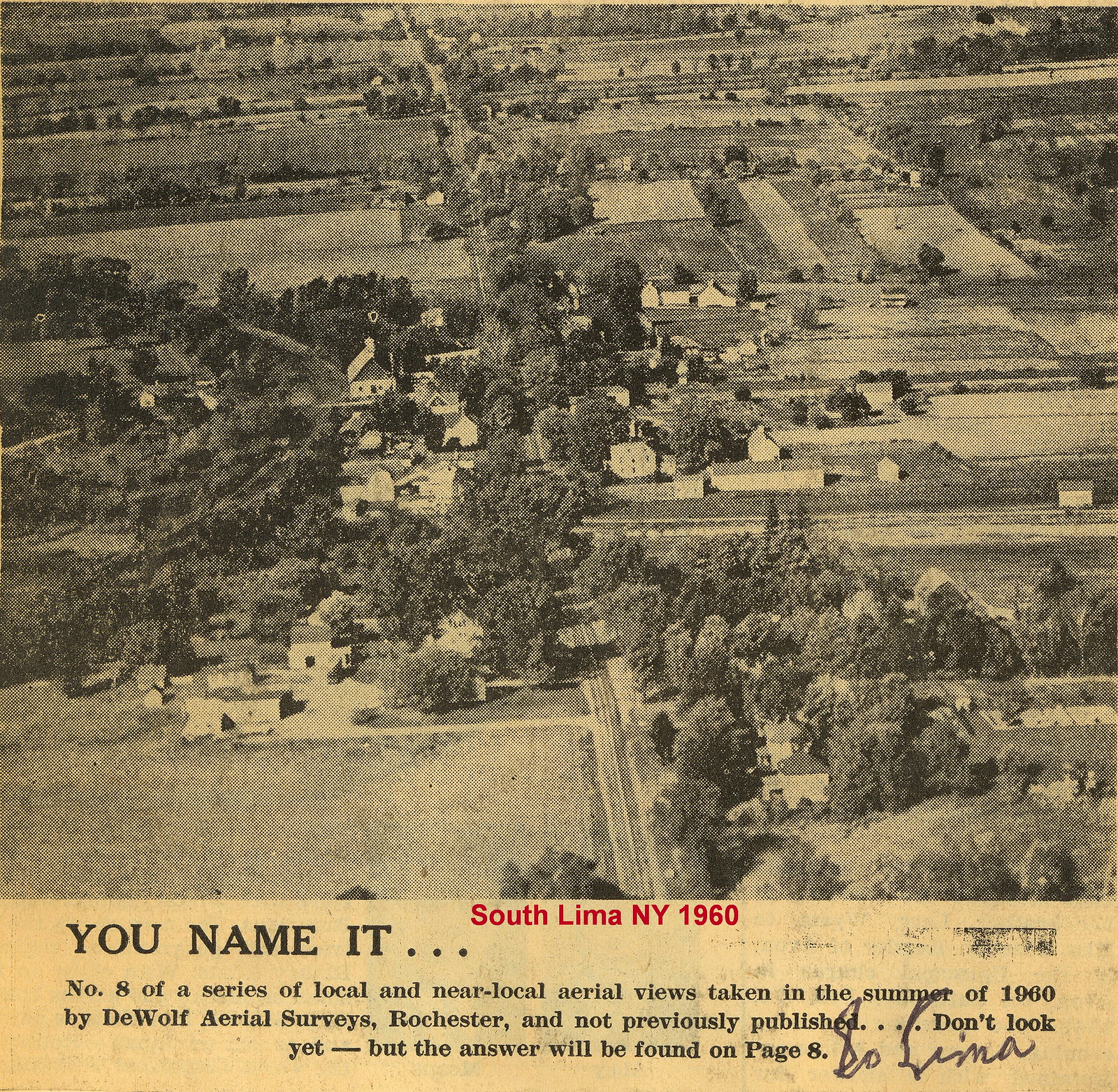The image appears to be an old photograph from the 1960s, likely scanned from an old newspaper or magazine. It shows an aerial view of South Lima, New York, as indicated by a red stamp at the bottom of the image. The photograph is black and white, capturing a large landscape featuring a small town with numerous houses, a main road running down the middle, several side roads, farmland, and an abundance of trees and clear areas. The overall print is grainy and dotted, characteristic of newspaper prints from that era, and the paper itself has yellowed over time. Beneath the photo, in small red text, it reads "South Lima, New York, 1960," followed by "You name it..." in larger letters, and "Number 8 of a series of local and near-local aerial views taken in the summer of 1960 by DeWolf Aerial Surveys, Rochester, and not previously published.... Don't look yet, but the answer will be found on page 8." Additionally, there appears to be a hand-written note, possibly a signature, in the bottom right corner, which is difficult to decipher but might say "So Lima" or "S. Lima."